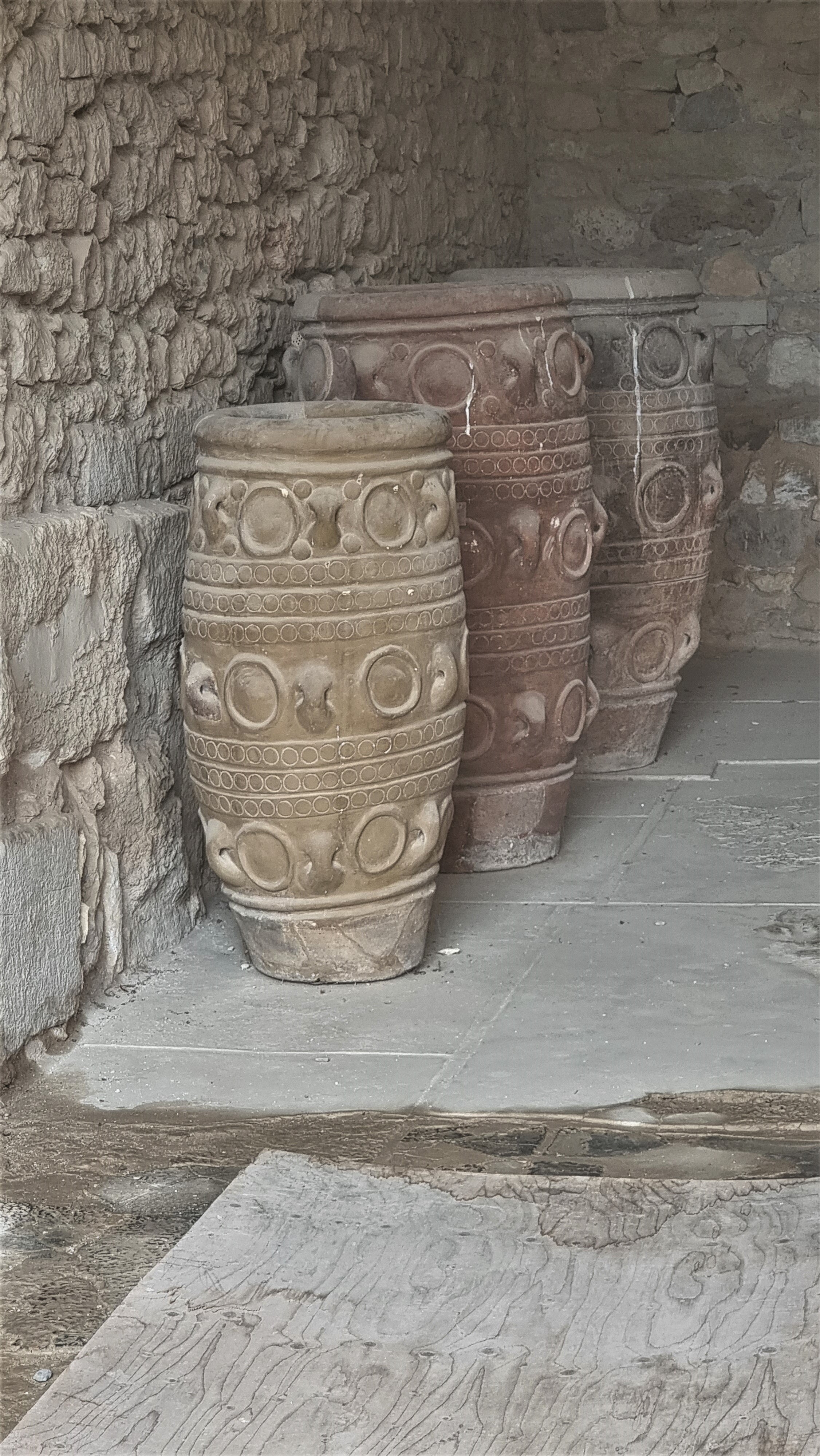The photograph captures an antiquated, dusty stone structure housing three intricately designed antique jars. The setting exudes a sense of ancient abandonment, with the stone walls showing rough, craggy texture and signs of wear. The jars themselves, layered with dust, each feature detailed geometric patterns. The frontmost jar is a small, light tan or golden yellow color, while the middle jar is larger and reddish. The largest jar, positioned at the back, has a muted grayish-blue hue. On the floor in the foreground lies a piece of wood amid the apparent grime of the dilapidated room, suggesting the area may have been affected by water damage. The overall lighting is dim, casting an aura of nostalgic eeriness over the scene, and highlighting the sense that this space is far removed from modern civilization.